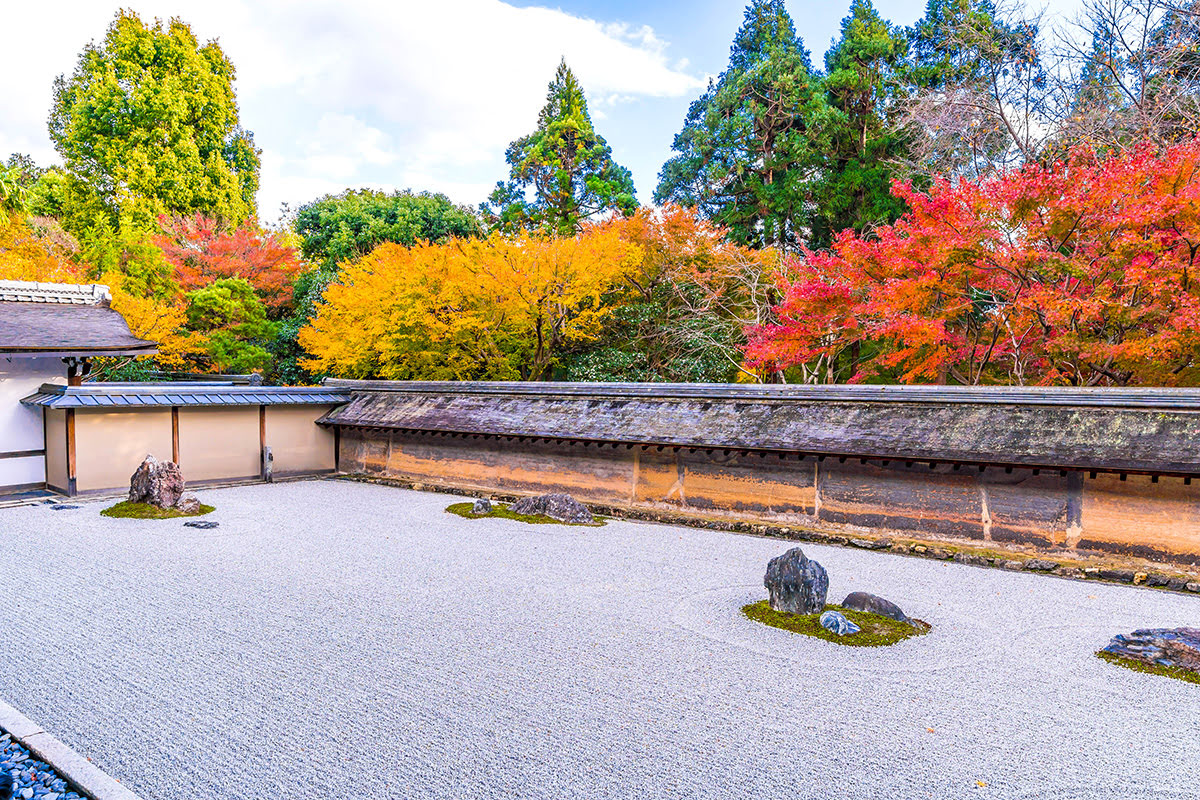The image depicts a serene rooftop Zen garden that exudes an Asian architectural influence. The garden is designed with a meticulous arrangement of gravel pathways and pebbles, interspersed with small boulders and neatly manicured grass patches. Traditional Japanese-inspired walls, characterised by their slanted roofs, border the garden and enhance its tranquil aesthetic. A variety of stones, some surrounded by moss, contribute to the garden's natural charm.

In the background, an array of trees in vibrant fall colors adds a picturesque quality to the scene. Prominent among these is a tree with a blend of red, orange, green, and yellow leaves, positioned slightly off the upper right corner. Adjacent to this tree stand tall green fir trees and a centrally located light green, almost yellow tree, all under a sky with white clouds in the back left. The background is further defined by a short wall that extends horizontally across the scene, intersected by another wall that creates a sense of depth and dimension. The garden floor, with its stone and gravel layout, appears almost like a carpet, contrasting with the organic nature of the trees and rocks. The overall composition showcases a beautiful, peaceful, and intricately detailed outdoor space that melds natural elements with architectural design.